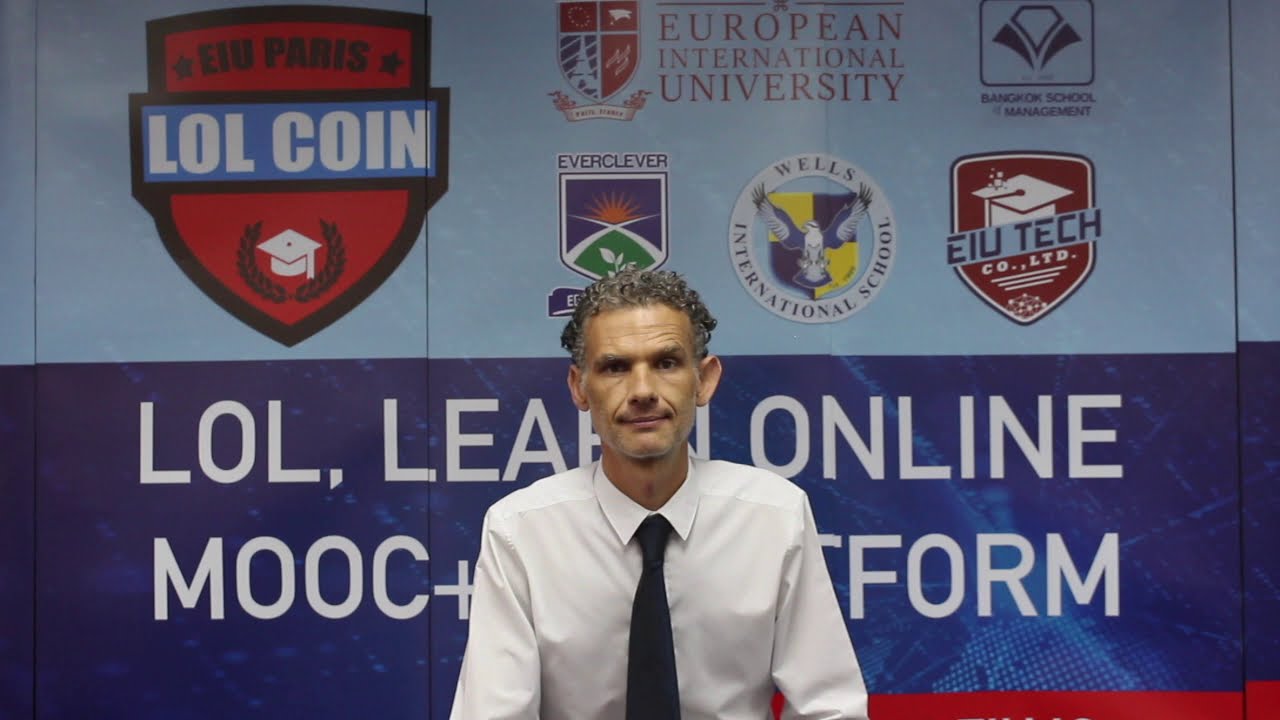This highly detailed photorealistic image showcases a man of apparent maturity, his salt-and-pepper curly hair and olive-toned skin lending him a distinguished appearance. He sports a white, long-sleeved dress shirt with a collar and a black tie, sitting upright and centered within the frame. The image captures him from the waist up, with his slightly protruding ears noticeable as he gazes directly into the camera.

Behind him is a vividly colored wall, split horizontally into a light blue upper half and a dark blue lower half. The top section of the wall features an array of logos and crests that suggest a scholarly environment, potentially a university forum or convention. On the left side, a prominent red crest with a blue banner bearing the words "LOL coin" is visible, accompanied by the label "EIU Paris" and an image of a graduation cap. The right side of the upper wall displays "European International University" in bold red letters surrounded by a collection of multicolored crests and logos in red, blue, green, yellow, and white. These include references to EIU Tech, Wells International School, and the Bangkok School of Management. Meanwhile, the underlying dark blue section of the wall is adorned with large white block letters that remain partially obscured by the man. This rich combination of visual elements strongly implies that the man is involved in an official academic capacity, potentially speaking or being photographed at an educational event tied to these institutions.